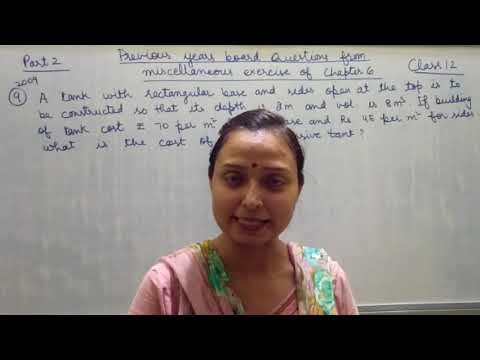This photograph captures a woman of East Indian descent with dark hair and skin, adorned with a traditional red bindi between her eyebrows. She is dressed in a vibrant pink blouse embellished with blue, white, and yellow floral designs around the collar area. Positioned centrally in the image, she gazes directly into the camera, appearing to be engaged in speaking, possibly conducting a class or presentation. She stands before a large, rectangular-shaped whiteboard that dominates the backdrop. The whiteboard features streaks running vertically and is bordered by a black frame on both the top and bottom edges. At the top of the whiteboard, handwritten text in blue ink includes a title centered on two lines, beneath which is a paragraph. Specific notations such as "Part 2" in the upper left corner and "Class 12" in the upper right corner are visible. The woman, smiling gently, adds a welcoming presence to the educational setting.